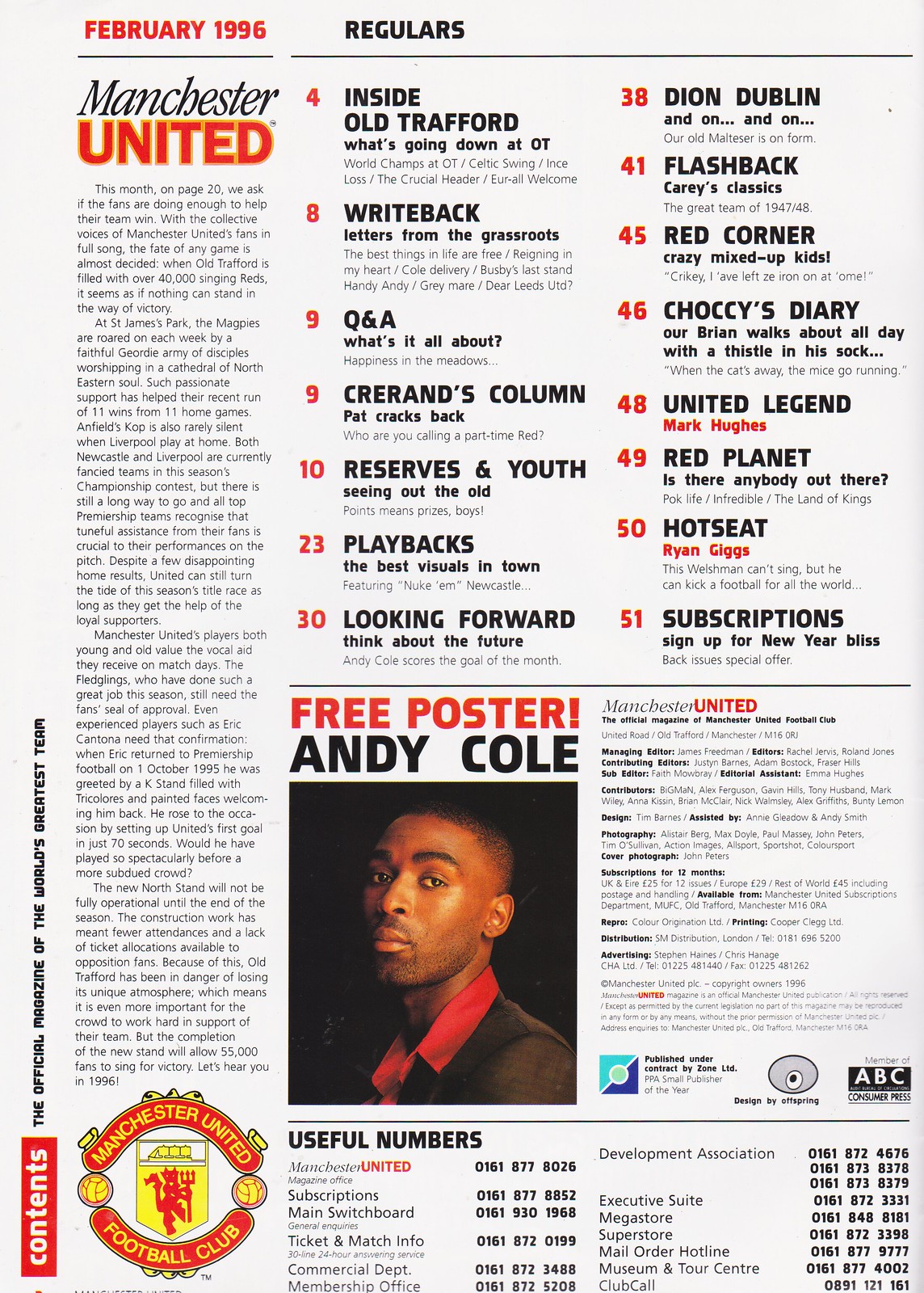The image captures a page from a magazine dated February 1996. It prominently features the Manchester United Football Club. In the top left corner, in red font, is the date "February 1996," adjacent to the word "regulars" in black. Below this, the heading "Manchester United" is displayed, with "Manchester" in black italics and "United" in bold red caps. The left column includes a detailed article about the club.

Toward the bottom left, the iconic Manchester United crest is visible, featuring a red devil with a pitchfork on a yellow background, the words "Manchester United" in yellow on a red background, and "Football Club" also in yellow on red.

The middle section of the page resembles a contents list, outlining various sections of the magazine with page numbers and headings in red and black font. These include:
- Page 4: Inside Old Trafford
- Page 8: Right Back
- Page 9: Q&A and Career Ads Column
- Page 10: Reserves and Youth
- Page 23: Playbacks
- Page 30: Looking Forward
- Page 38: Dion Dublin
- Page 41: Flashback
- Page 45: Red Corner
- Page 46: Chalky's Diary
- Page 48: United Legend
- Page 49: Red Planet
- Page 50: Hot Seat
- Page 51: Subscriptions

At the bottom center, there's an image of a black man in a suit or blazer with a red collared shirt, looking directly at the camera. Above his image, the text "Free Poster Andy Cole" is split into "Free Poster" in red and "Andy Cole" in black. Beneath this, a section labeled "Useful Numbers" provides various mailing and subscription contacts. The background of the page is predominantly white with black text, adding a clean and readable aesthetic.